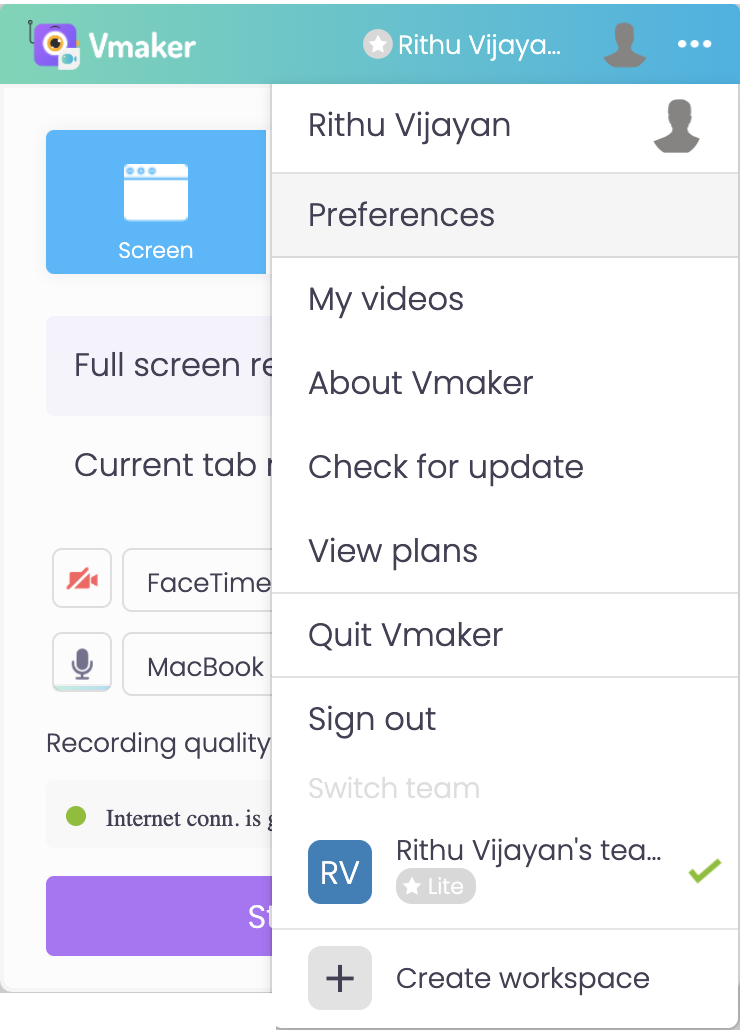The image is a vertically rectangular screenshot, likely taken from a cell phone. It prominently features an active pop-up window on the right that partially obscures the main content of the screen. The visible upper-left corner of the main screen displays the "V-maker" logo, followed by the user name "Rithu Vijayan," spelled out as R-I-T-H-U V-I-J-A-Y-A-N. 

The pop-up window on the right side of the image lists several menu options in a vertical format. These options are: "Preferences," "My Videos," "About V-maker," "Check for Update," "View Plans," "Quit V-maker," "Sign Out," and "Switch Team." 

At the bottom right of the screen, next to the pop-up, there is a plus button with the label "Create Workspace."

In the partially visible section of the main screen to the left, there is a blue button labeled "Screen." Below this button, there is an option for "FaceTime or MacBook" selection, followed by a setting for "Recording Quality." However, only the left portion of these elements is visible due to the overlay of the pop-up window.